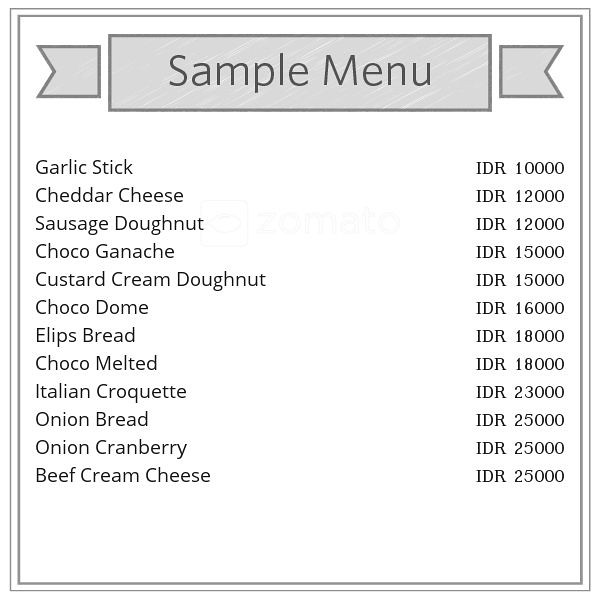The image is a black-and-white graphic design displaying a sample menu, which is framed by a subtle black border. At the very top center, inside a horizontal rectangle flanked by makeshift ribbon-like decorations on each side, the words “Sample Menu” are prominently displayed in black font. The menu features various items listed vertically from top to bottom with their corresponding prices in Indonesian Rupiah (IDR). The items and their prices are as follows: Garlic Stick (10,000 IDR), Cheddar Cheese (12,000 IDR), Sausage Donut (12,000 IDR), Choco Ganache (15,000 IDR), Custard Cream Donut (15,000 IDR), Choco Dome (16,000 IDR), Ellipse Bread (18,000 IDR), Choco Melted (18,000 IDR), Italian Croquette (23,000 IDR), Onion Bread (25,000 IDR), Onion Cranberry (25,000 IDR), and Beef Cream Cheese (25,000 IDR). All the text is in black on a white background, providing a clear and concise layout of the menu items and their prices.